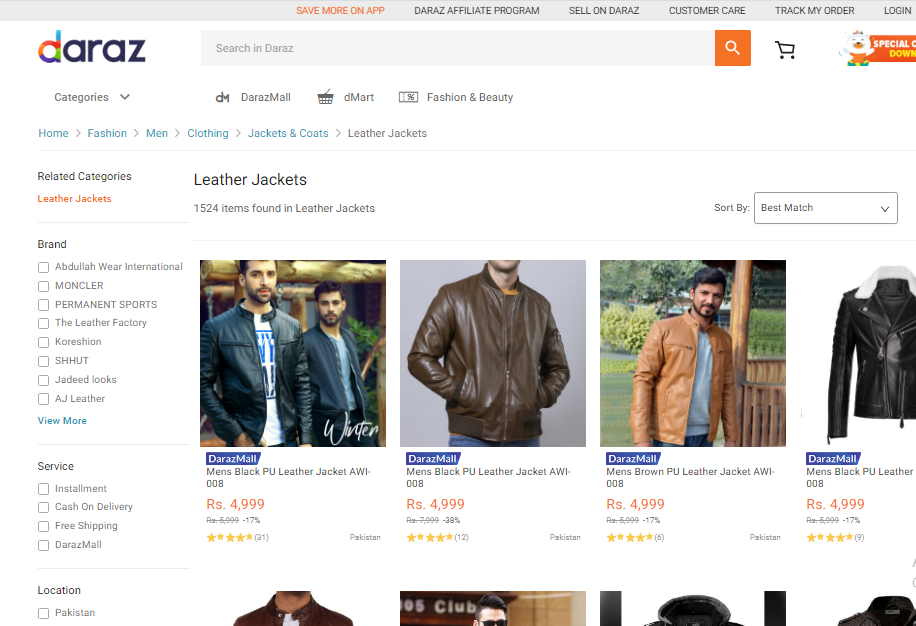This image displays an online shopping page from Daraz, a well-known e-commerce platform. The Daraz logo features a distinctive multicolored "D" in shades of purple, red, orange, yellow, and green, while the remaining letters "A-R-A-Z" are in black. The page is geared towards men's fashion. At the top, in vibrant orange text, there is a promotion encouraging users to "Save More on App." Additional navigation options include "Daraz Affiliate Program," "Sell on Daraz," "Customer Care," "Track My Order," and a prompt to "Log On." Below this section is a search bar framed with an orange square housing the search icon, along with a shopping cart icon.

The page predominantly features leather jackets, indicating a focus on trendy menswear. The first visible row includes two men modeling jackets. Both jackets appear to be on sale. The second man in the first row wears a black PU leather jacket. Beside him, a bearded man with a mustache is modeling a tan jacket. The last jacket in this row is a black PU leather jacket with a somewhat contrasting white collar.

The second row of images is partially cut off, revealing only glimpses of the menswear, making it difficult to discern specific details. Overall, the page emphasizes a variety of stylish leather jackets available for purchase.